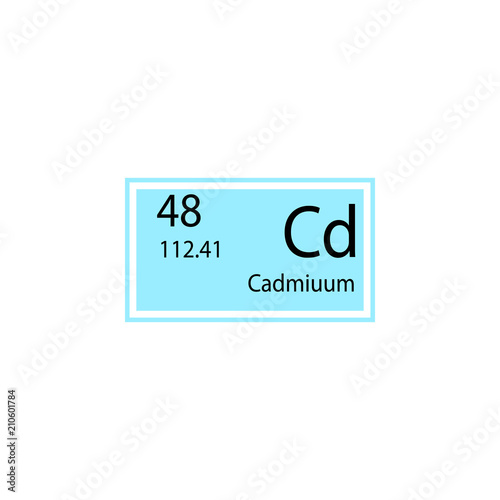The image is a detailed stock graphic depicting an element from the periodic table, specifically cadmium. Centered on a white background is a horizontally oriented, light blue (teal) rectangle bordered by white, and then again by the same light blue. In the upper left corner of this rectangle is the atomic number "48" in black text, and directly below it, in smaller black text, is the atomic weight "112.41". On the right side, prominently displayed in large black font, is the chemical symbol for cadmium, "Cd" (with a capital 'C' and a lowercase 'd'). Below this symbol, still on the right side and in smaller black font, is the full name of the element, "cadmium". Additionally, on the left edge of the white background, text runs vertically, stating "Adobe Stock" followed by a gray line and the reference number "#210601784" in gray.